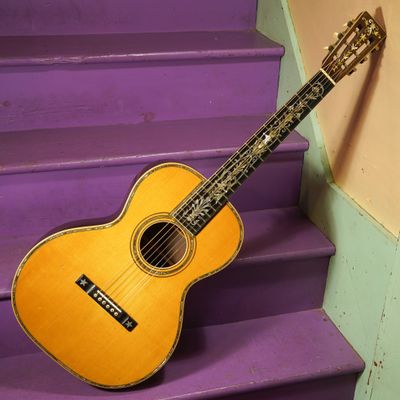The image features a slightly worn, small wooden guitar with a golden finish sitting on vibrant, bright purple-painted wooden steps, which show signs of use with mud stains. The guitar, adorned with a gold embellishment resembling a fleur-de-lis design running along its neck, leans against a teal blue wall that transitions to an orange-brown color above. The surrounding wall shows wear with noticeable splatter marks, indicating its location is likely an outdoor staircase, possibly leading to an apartment complex. The scene is lit well enough to cast the guitar's shadow, highlighting the contours and textures of both the guitar and the rugged steps.